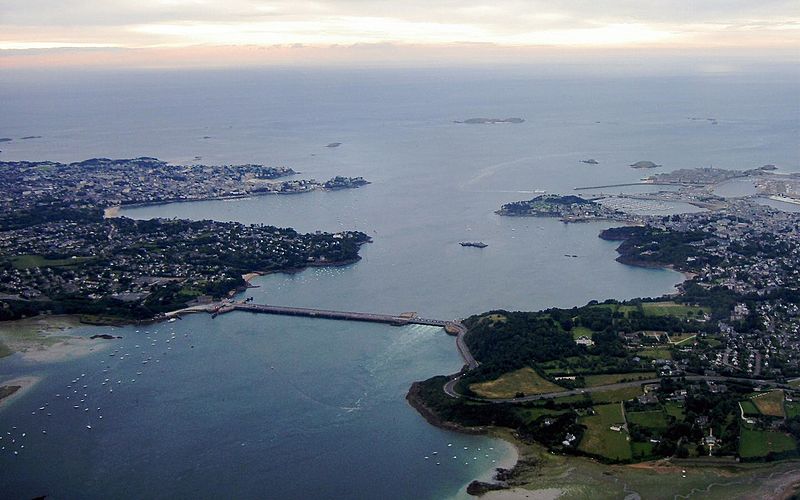This is a color aerial photograph taken during the daytime, showcasing an expansive view of two lush, green islands connected by a substantial concrete bridge. The islands are separated by vibrant blue water, dotted with several boats and smaller islets. The island on the left takes up a considerable portion of the image, characterized by dense vegetation and forestry areas, with a noticeable concentration of buildings towards the right side, suggesting a populated area. In contrast, the island on the right features fewer trees and predominantly consists of residential houses and buildings. The sky above displays a beautiful blend of colors, suggesting either sunrise or sunset, with shades of gray, yellow, and pink hues highlighting the partially cloudy sky. A dock is visible on the right-hand side, indicating the presence of maritime activities. The bridge, a long gray structure, seamlessly connects the two landmasses, facilitating transportation across the picturesque body of water.